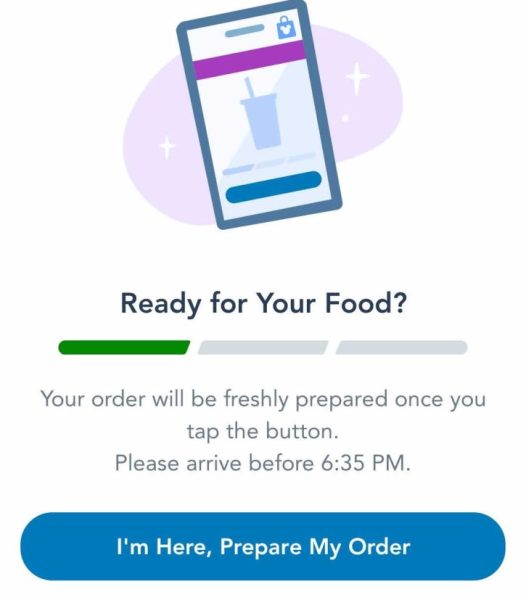**Detailed Caption:**

On a clean, white background, there's a light purple, circular blob adorned with various star signs. Below this celestial design, there's an illustration depicting a smartphone. On the smartphone screen, icons of a shopping bag and a cup with a straw are prominently featured. At the bottom of the phone's display is a blue button. Beneath the smartphone illustration, the phrase "Ready for your food" is clearly written.

Further down, to the left, there's a green bar, accompanied by two gray bars to its right. Dropping a line below this, there's a message stating, "Your order will be freshly prepared once you tap the button. Please arrive before 6:35 PM." There's a line break below this text, revealing a large, dark blue, elongated rectangular button with the phrase "I'm here preparing my order" written in white text in the center.

The remaining area of the image consists of a vast expanse of white, empty space.